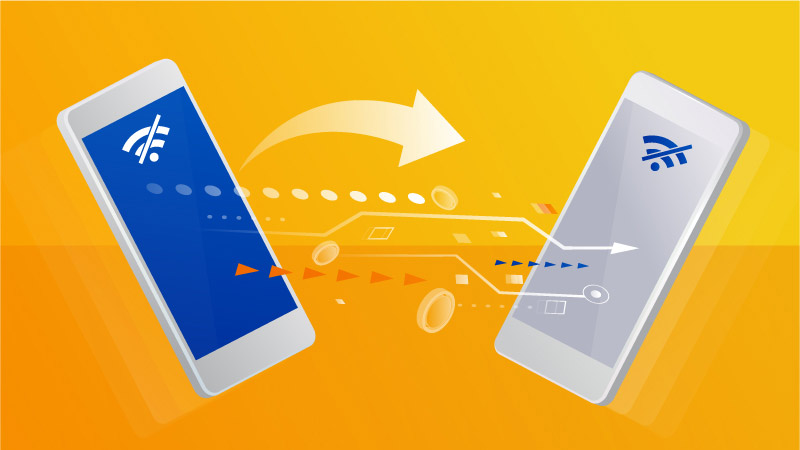This digitally created image is a cartoon-style illustration featuring two smartphones against a two-tone orange background, where the top half is light orange and the bottom half is dark orange, separated by a solid white line. The phone on the left has a blue screen with a white Wi-Fi symbol crossed out by a diagonal line, and the phone on the right has a gray screen with the same Wi-Fi icon also crossed out. Various arrows and dots in white, yellow, and orange travel from the left phone to the right, implying the transfer of information between the devices. The overall color palette includes shades of gray, blue, yellow, orange, and white, enhancing the instructional vibe of the image, potentially indicating a guide for troubleshooting or connecting smartphones.